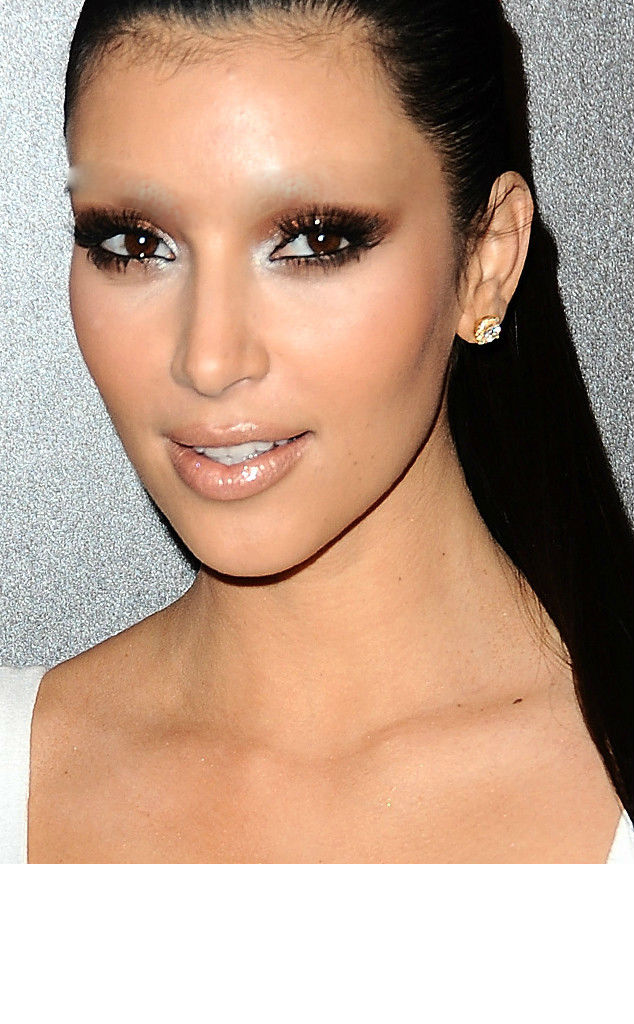In this photograph of a woman, we see her from the upper chest to her forehead, with the top of her head and the rest of her body out of frame. The woman is wearing a low neckline white top, although it's unclear whether it is a shirt or a dress. Her long black hair cascades over her left shoulder, which appears on the right side of the image. She is adorned with a gold stud earring featuring a white diamond in the center, resembling a flower. Her lips are pink, possibly enhanced with lip gloss or lipstick. She has large black eyelashes and brown eyes that look straight ahead, as does her face. Notably, her eyebrows are missing. The background is a grayish silver color, adding a neutral contrast to the beige-tan tones of her skin. The overall scene suggests that she could be a famous person having her portrait taken, given the carefully arranged elements and her poised expression.